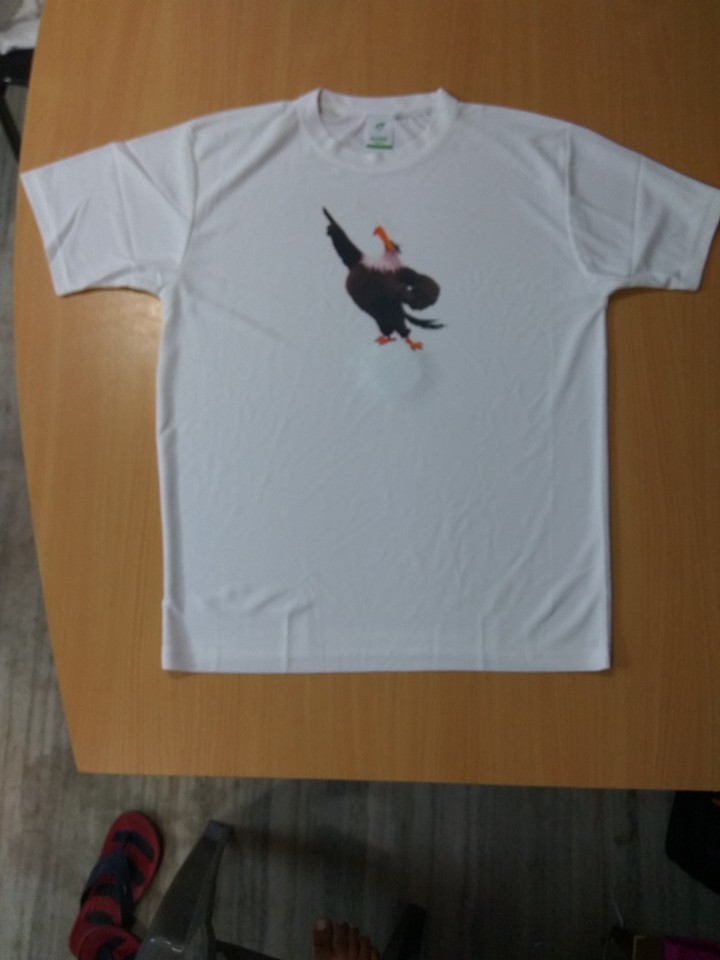This is a top-down photograph of a white short-sleeved t-shirt laid out on a light brown, rectangular table with tapered edges. The t-shirt features a detailed illustration of a rooster with distinctive dark chocolate brown feathers and a white head and neck. The rooster's beak and feet are bright orange, and it has a small, wispy brown tail feather. The rooster is depicted with one wing pointed straight up and the other resting on its hip, while its chest is puffed out prominently. At the top of the shirt, there is a white tag with lime green writing and a lime green symbol.

The table is set against a flooring that mimics the appearance of light brown and tan wood. In the bottom-left corner of the photograph, there is a right foot with white nail polish and part of a black leg of a chair visible. Also on the table, near the edge, lies a pair of flip-flops that are mostly red with black stripes on the soles and black straps. The t-shirt itself shows slight wrinkling at the bottom edge, the sleeves, and the shoulder area.